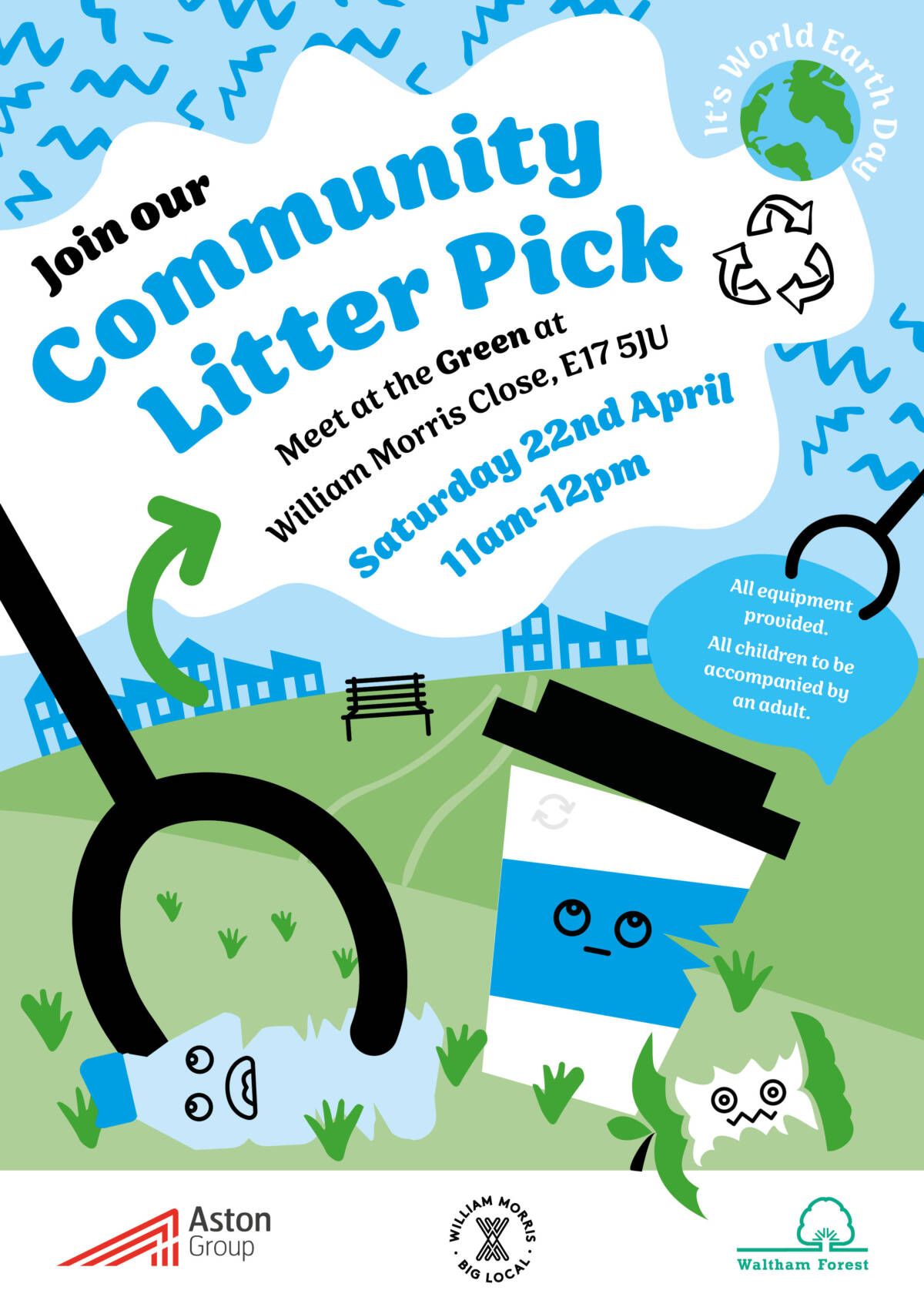This vibrant poster invites the community to join a litter pick event. Against a backdrop of a light blue sky with squiggly lines representing birds, the poster features a green field scattered with lively, anthropomorphic trash, including a plastic bottle, a cardboard coffee cup with a blue stripe, and a sickly-looking apple core—each with expressive faces and eyes. At the center, a black grabber with a horseshoe-shaped head reaches down to pick up the trash. The text, set against a white cloud near the top, reads: "Join our community litter pick. Meet at the green at William Morris Close, E17 5JU, Saturday 22nd April, 11 AM to 12 PM." In the upper right, a recycling symbol intertwined with three arrows and an image of the Earth proclaims, "It's World Earth Day." The bottom of the poster features various sponsor logos, supporting this environmentally conscious event.